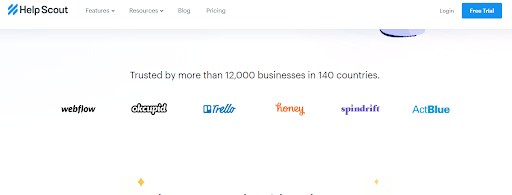The image displays a webpage with a clean, white background. In the top-left corner, the logo "Help Scout" is prominently featured, with "Help Scout" written in black text next to an icon consisting of three blue, diagonal lines slanting to the right. Across the top of the page, there are several navigational tabs starting from the left: Features, Resources, Blog, and Pricing. On the top right, there are options to log in and a prominent blue button labeled "Free Trial."

Dominating the center of the webpage, a bold black text states, "Trusted by more than 12,000 businesses in 140 countries." Below this statement, six business names are displayed in a horizontal layout. From left to right, the businesses listed are:
1. Webflow, written in black.
2. Occupied, written in white with a black outline.
3. Trello, written in blue.
4. Honey, written in orange.
5. Spintrift, written in purple.
6. ActBlue, written in blue.

The overall layout is clean and professional, emphasizing the credibility and wide usage of Help Scout across various businesses worldwide.